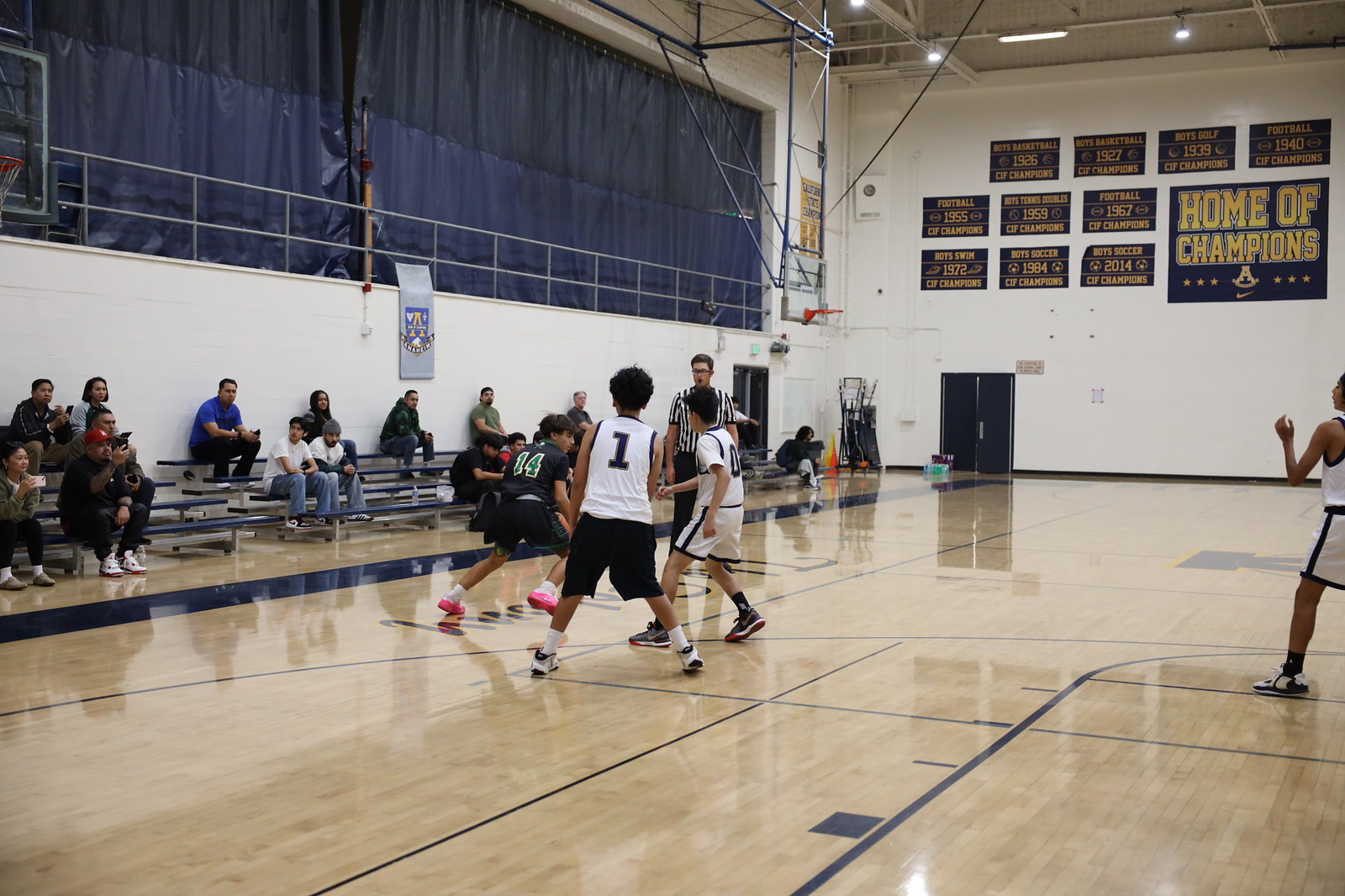The image shows a high school basketball game taking place in a large gymnasium. On the court, there are four players: one in a black uniform and three in white uniforms. Referee in a striped shirt is visible, indicating the game is in progress. The far back wall features several banners, with a prominent one reading "Home of Champions," listing years from 1926 to 2014, adorned with blue flags and gold text. On the left side, about 15-20 spectators are seated across three rows of bleachers, with a white wall behind them and a metal barrier topped with a blue curtain. The spectators seem engaged, watching the game unfold.